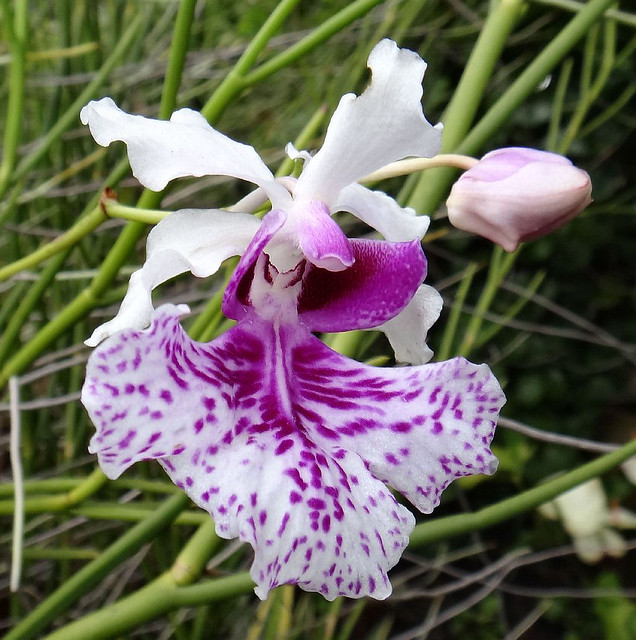This close-up photograph taken outdoors captures a striking Vanda tricolor orchid in its full splendor. The flower is centrally positioned and in sharp focus, showcasing its star-shaped arrangement of four to five curvy white petals. The standout feature of this orchid is the large, fan-shaped petal at the bottom, which exhibits a beautiful blend of colors – it starts pink at the base and transitions to white with whimsical purple spots and lines emanating outward, resembling an intricate webbing. To the right of the main flower, an unopened bud hints at the flower's continued bloom. The background is a soft blur of thick green stems and yellowish branches, devoid of any other plants, animals, or text, which enhances the vivid details and delicate beauty of the orchid.